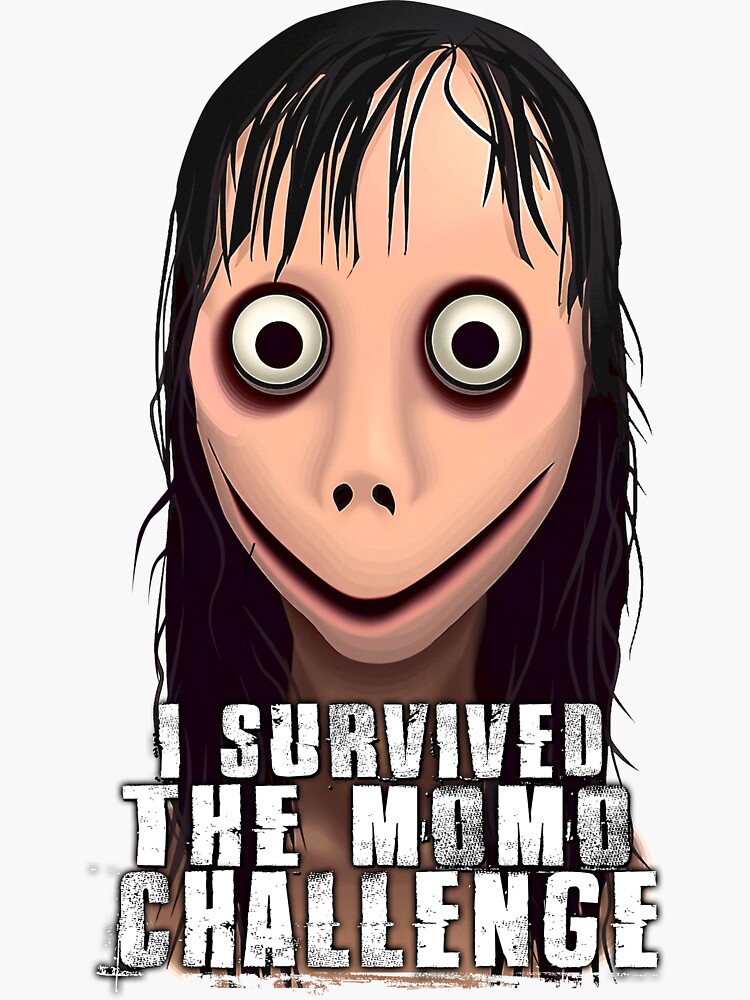This is a detailed computer-generated image with a white background, prominently featuring an unsettling cartoon character often associated with the "Momo challenge." The character's face is pallid and ghastly, with straggly, oily black hair falling in short bangs across the forehead and longer, stringy strands on the sides. The large, bulging eyeballs have jet black pupils framed by dark red bags, creating a haunting stare. The figure lacks eyebrows and has a nose reminiscent of Lord Voldemort's, marked only by two dark holes. Its unnaturally stretched, toothless smile forms a sharp V-shape that extends up the sides of the cheeks, giving an appearance as if the mouth has been grotesquely sliced open. The character's neck is elongated and thin, leading to a bare chest. Superimposed on the image are the words "I survived the Momo challenge," written in a horror-themed font with intermittent black speckles and squiggly distortions, adding to the unnerving atmosphere of the image.